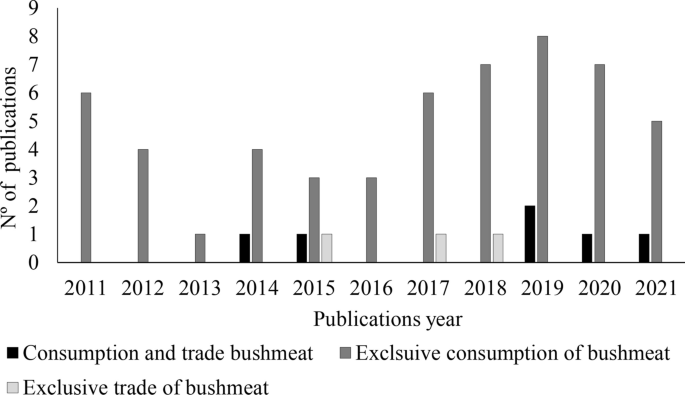This image features a detailed bar chart with three distinct shades: black, dark gray, and light gray, all set against a white background. The vertical axis on the left side marks the number of publications, ranging from 0 to 9, while the horizontal axis spans the publication years from 2011 to 2021. Each year displays up to three bars representing different categories: black bars for "Consumption and Trade of Bushmeat," dark gray bars for "Exclusive Consumption of Bushmeat," and light gray bars for "Exclusive Trade of Bushmeat." The chart's legend at the bottom clarifies these color codes. Notably, some years, such as 2011 and 2012, only feature dark gray bars, while 2015 is unique with all three bar types present. In 2019, the dark gray bar peaks, indicating the highest number of publications on exclusive bushmeat consumption, reaching up to 8. Exclusive trade of bushmeat is only noted in the years 2015, 2017, and 2018.